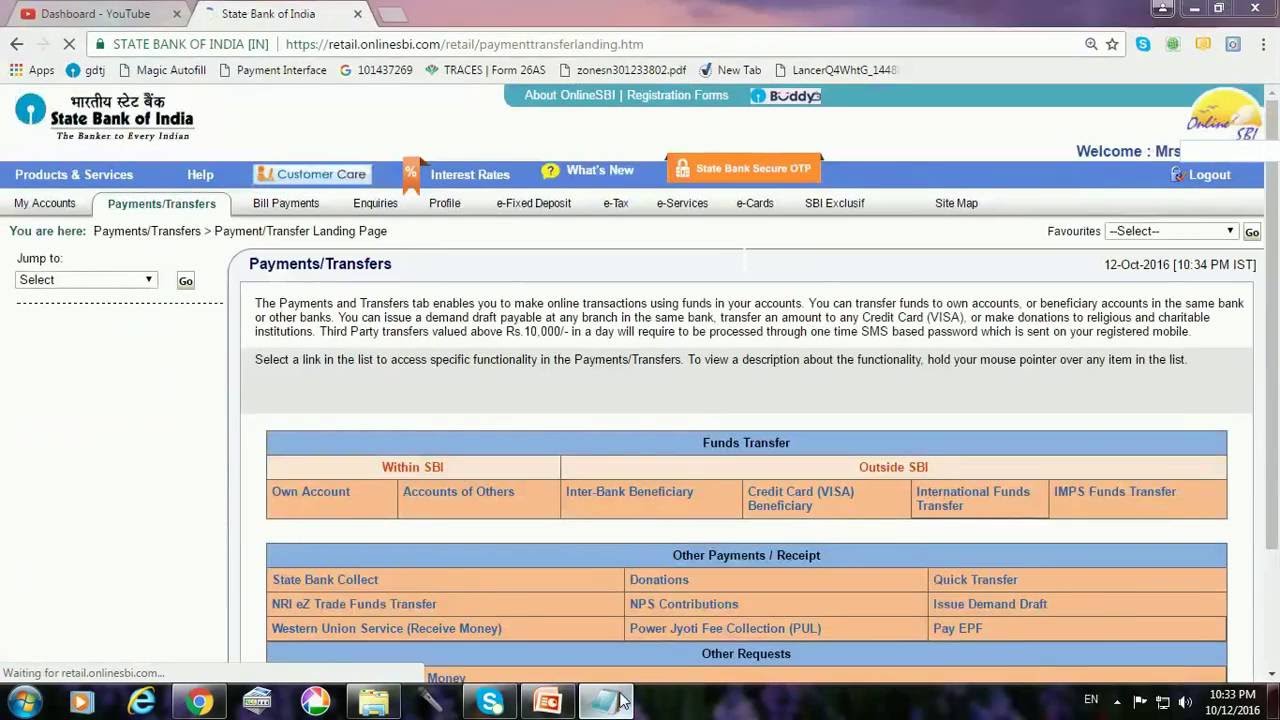The image depicts a detailed bank statement from the State Bank of India, likely belonging to an individual. At the top of the statement, a dark blue header features several navigational options: "Products and Services," "Help," "Customer Care," "Interest Rates," and "What's New." Additionally, there is a lock icon next to the label "Bank of India," which is somewhat difficult to read.

Below this, a white header contains more navigation tabs including "My Accounts," "Payments," "Transfers," "Bill Payments," and an additional "Help" option at the end. Centrally displayed is a prominent section titled "Payments and Transfers," which provides information on online transactions using the user's account funds. It offers a detailed explanation that these funds are accessible for various online transactions.

The document is dated October 12, 2016. Directly underneath, the section labeled "Funds Transfer" appears highlighted in blue, with the associated details in orange, thus standing out clearly. Another similar section also shows transaction details with blue headers and orange text. At the bottom, a black strip features computer-related icons, providing additional functionality or quick access options.